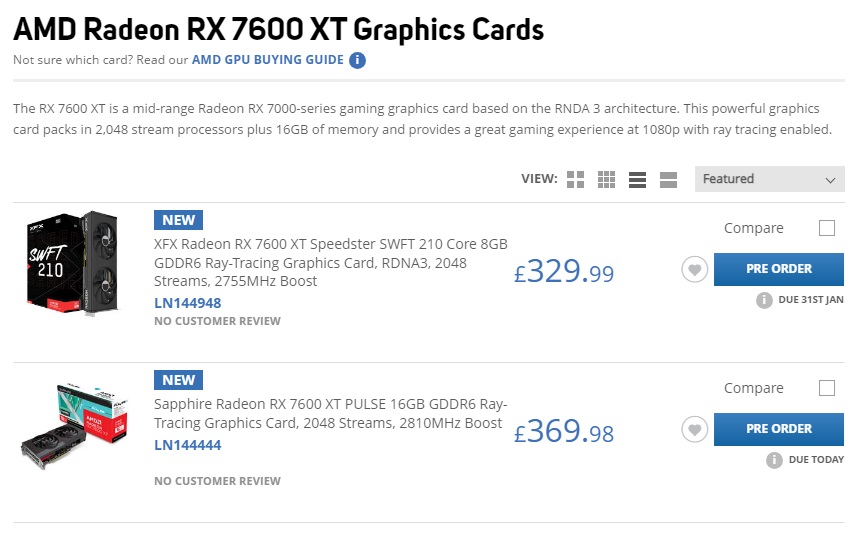The image prominently displays the header "AMD Radeon RX 7600 XT Graphics Card" in the top left corner. Just below this, there's an informative suggestion, "Not sure which card? Read our AMD GPU buying guide," accompanied by a circular icon containing the letter 'i'. 

The main body of text describes the RX 7600 XT, detailing it as a mid-range gaming graphics card in the Radeon RX 7000 series, leveraging the advanced RDNA 3 architecture. It boasts 2,048 stream processors and 16GB of memory, offering an excellent 1080p gaming experience with ray tracing enabled.

Lower down, the image showcases two products:

1. On the left, the "XFX Radeon RX 7600 XT Speedster" is listed with a price of $329.99.
2. Below it, the "Sapphire Radeon RX 7600 XT Pulse" is priced at $369.98.

To the right of each product listing, there is a heart symbol, followed by the word "Pre-Order" enclosed in brackets.